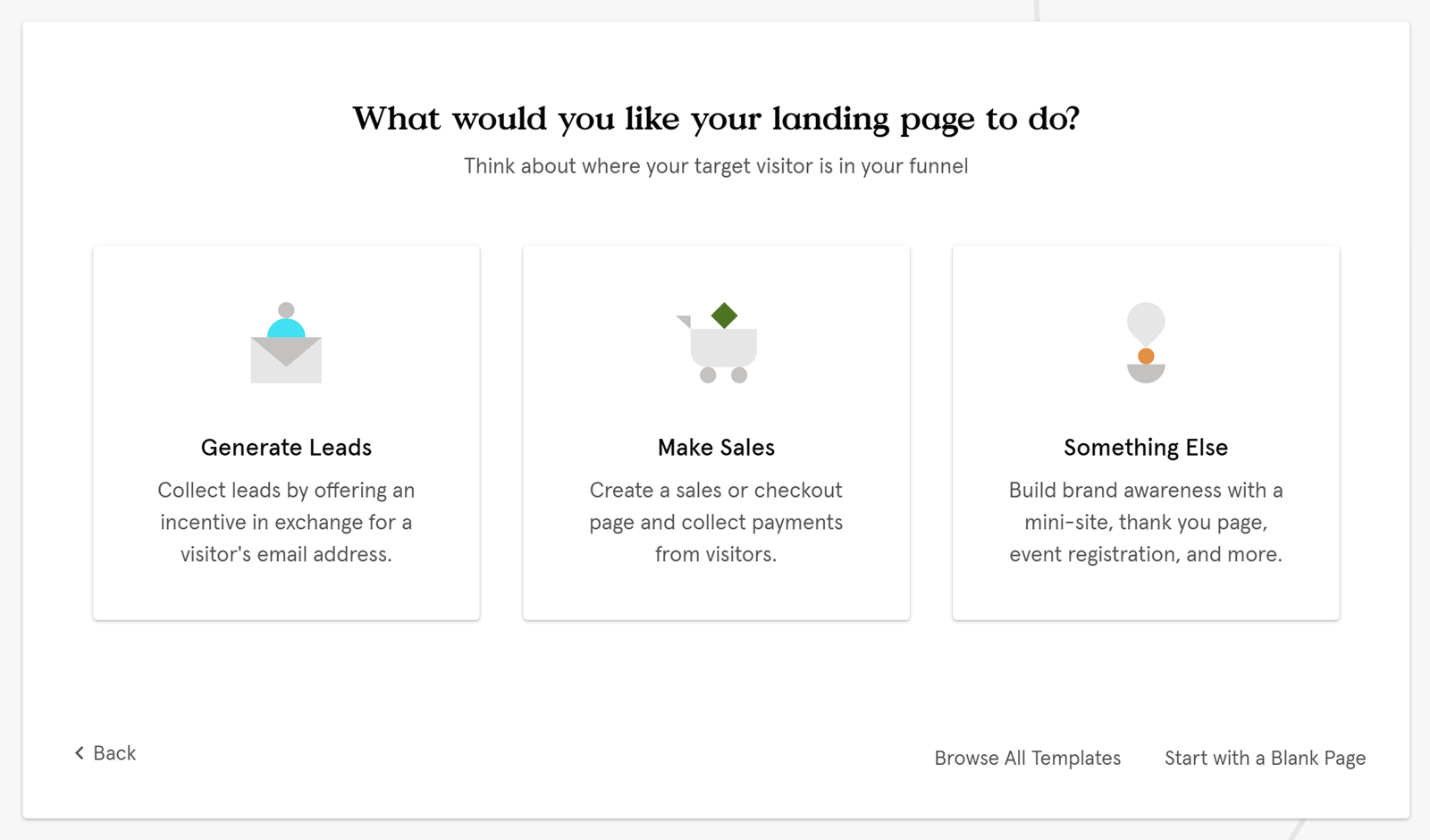This image features a clean, white background with a lighter gray border encircling it. Dominating the top center of the image is a thought-provoking question in bold text: "What would you like your landing page to do? Think about where your target visitor is in your funnel." 

Directly beneath this header are three equally sized squares arranged in a horizontal line, each containing distinct icons and informative text.

1. **Left Square**: 
   - **Icon**: An envelope with a person emerging from it.
   - **Title**: Generate Leads
   - **Description**: Collect leads by offering an incentive in exchange for a visitor's email address.

2. **Middle Square**: 
   - **Icon**: A shopping cart with a diamond atop it.
   - **Title**: Make Sales
   - **Description**: Create a sales or checkout page and collect payments from visitors.

3. **Right Square**: 
   - **Icon**: A small boat with a circular object and a balloon above it.
   - **Title**: Something Else
   - **Description**: Build brand awareness with a mini-site, thank you page, event registration, and more.

The rest of the image is largely blank white space, emphasizing the text and icons in the center. At the very bottom of the page, the lower left corner features a small arrow accompanied by the word "Back," suggesting a navigation option to return to a previous page. Meanwhile, in the lower right corner, there are two prompts: "Browse All Templates" and in the very bottom right corner, "Start with a Blank Page," both inviting the user to explore further options for their landing page design.

Overall, the image serves as an engaging guide, offering clear options for tailoring a landing page based on specific objectives.